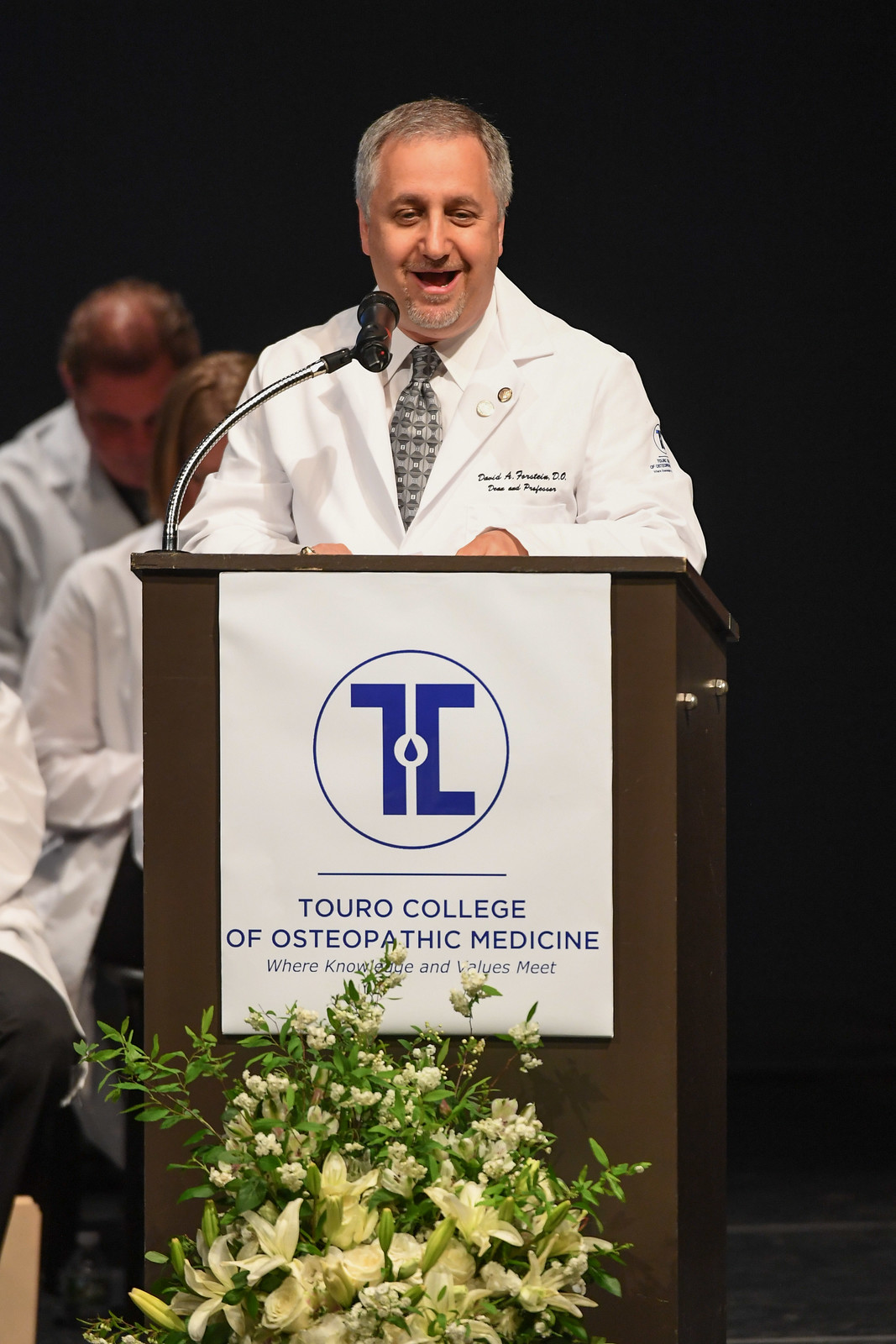A man, presumed to be a doctor, is depicted in this detailed image giving a speech at a wooden podium adorned with a white banner and a bouquet of white lilies and other flowers. The banner features the logo and text of Touro College of Osteopathic Medicine, where the institution's tagline reads, "Where Knowledge and Values Meet," in blue text against a white background. The man has grayish-brown hair, a goatee, and wears a white medical jacket with a black-and-white tie. His jacket displays a monogram, although it is difficult to read clearly. He is smiling while speaking into the microphone, and several other individuals in white lab coats are seated behind him, watching attentively. The scene is primarily dark in the background, drawing attention to the speaker and his colleagues on stage.